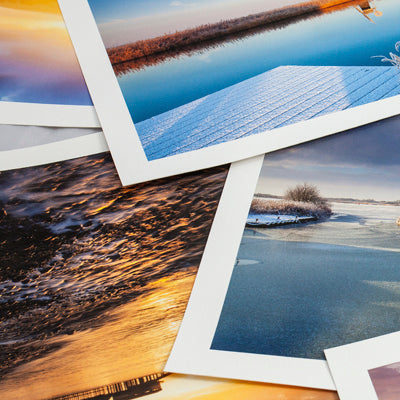This is a color photograph that appears to be a close-up compilation of five other nature-themed photographs, scattered and laid out on a table. Each individual photo within the collection features a white border, giving the impression they were printed at home. The bottom-left photo showcases an ocean scene tinged with yellow-orange hues, possibly capturing a sunset. Above this is another image with a portion of a lake or ocean, visible in the upper right but only partially due to the overlapping arrangement. Toward the lower right, there's a small fraction of another photo, mostly showing its white frame. The most prominent and visible photo is in the upper right corner, displaying a body of water, perhaps a lake or pond, set against a sky. Collectively, these photos present a vivid palette of yellows, pinks, blues, and earthy browns, capturing serene moments of nature with beach and water themes, all laid out on a tan background that enhances their colorful, clean aesthetic.